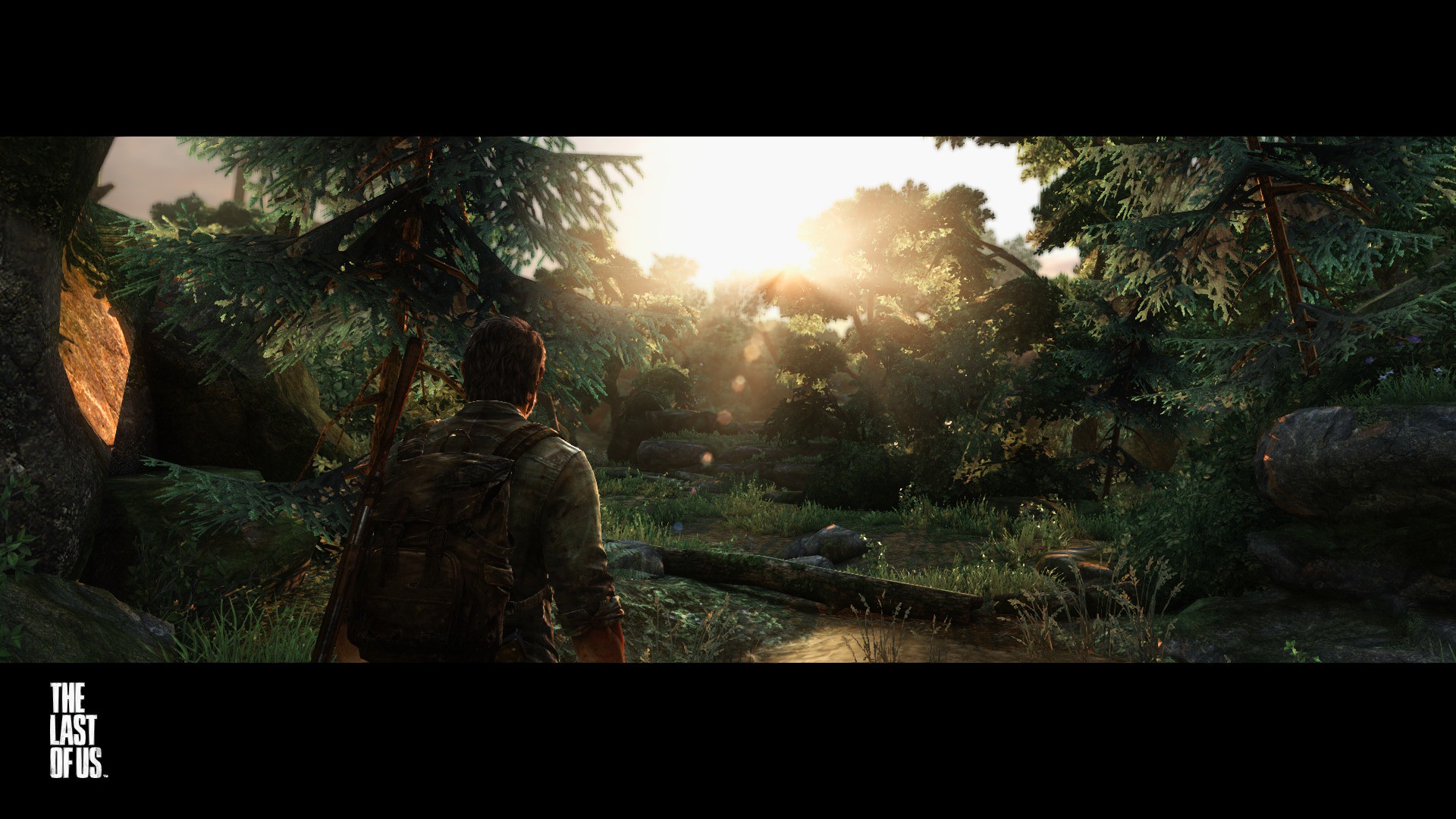This image is a color screenshot from the video game "The Last of Us." It features a cinematic widescreen format with large black bars at the top and bottom. In the bottom left corner, within the black bar, the game title "THE LAST OF US." is displayed in bold white capital letters. The scene depicts a lush, dense forest with numerous tall evergreen trees and a fallen log in a small clearing. The sun is either setting or rising, positioned at the center top, casting bright yellow sunspots and a lens flare throughout the middle of the image. In the foreground, the protagonist Joel Miller stands with his back to the viewer. He is dressed in dark, dingy clothing, including a denim jacket with rolled-up sleeves. He has short brown hair and a dark backpack, to which a hunting rifle is attached on the left side. The atmospheric lighting and detailed environment create a vivid, immersive scene characteristic of the game's aesthetic.